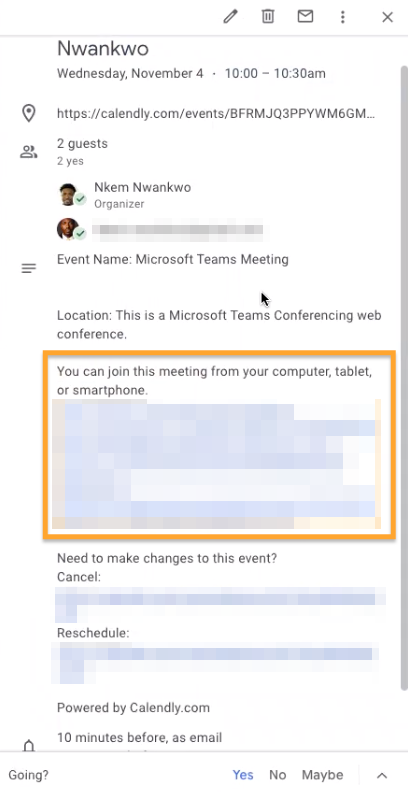A screenshot captured from a smartphone displays an invitation for a meeting. At the top, the heading features the last name "Nuankwo," identifying the creator of the meeting. Scheduled for Wednesday, November 4th, from 10:00 to 10:30 a.m., the invitation includes a web address for the virtual gathering via Microsoft Teams. It notes that two guests have confirmed their attendance.

The meeting organizer is listed as Nakem Nuankwo, and the invitee's name is blurred out for privacy. The event is titled "Microsoft Teams meeting," and the location is specified as an online conference accessible through a computer, tablet, or smartphone.

Instructions for changes to the event are provided, with links available for canceling or rescheduling the meeting. The footer of the invitation indicates it's powered by Calendly.com, although the full text is partially cut off. At the bottom, recipients are prompted to respond with their attendance status—Yes, No, or Maybe.